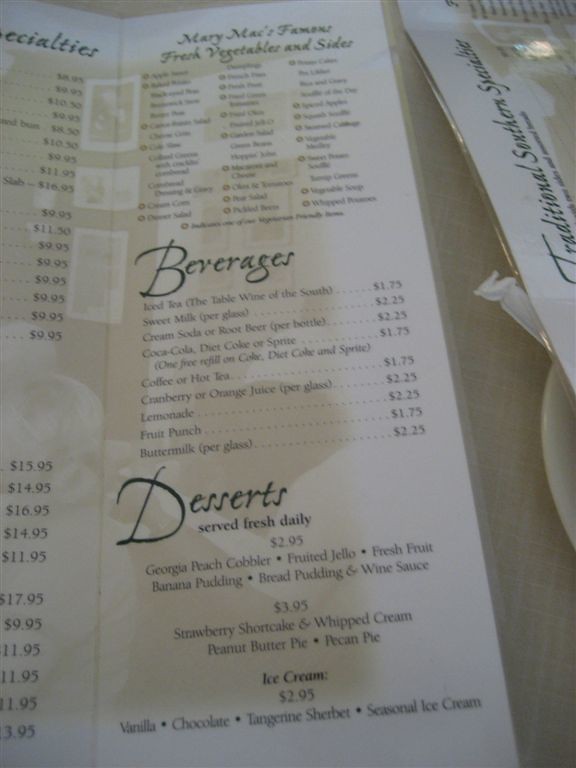The image depicts a laminated white menu placed on a beige tablecloth with another identical menu positioned to the right. Although the picture is somewhat unclear, the details of the menu are discernible. The menu text is superimposed on a blurred background image, possibly showcasing the restaurant's interior ambiance. 

At the top of the menu, the heading reads "Mary Max," followed by "Famous French Fresh Vegetables and Sides," as well as sections for "Beverages and Desserts." The adjacent menu to the right displays the heading "Traditional Southern Specialties." 

The menu is printed in black ink and lists several food and drink items along with their prices. For desserts, options include:

- Georgia Peach Cobbler
- Fruit Jello
- Fresh Fruit
- Banana Pudding
- Bread Pudding with Wine Sauce ($2.95)
- Strawberry Shortcake with Whipped Cream
- Peanut Butter Pie
- Pecan Pie ($3.95)
- Vanilla, Chocolate, and Tangerine Sherbet
- Seasonal Ice Cream ($2.95)

The detailed descriptions and pricing provide a glimpse into the Southern-inspired offerings of the establishment.